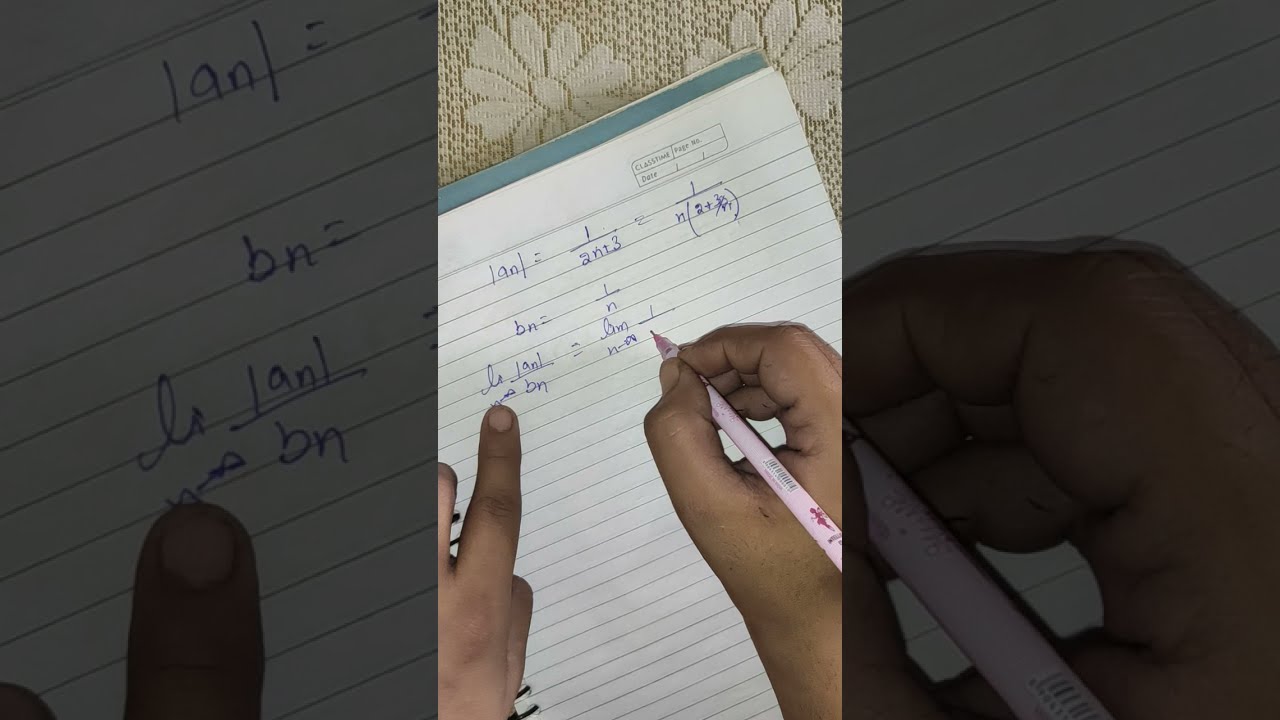This photograph captures an intricate study scene set against a lace, floral-patterned tablecloth. In the center, a ruled notebook tilted to the left reveals someone deeply engaged in solving mathematical equations, likely algebra or calculus, characterized by the presence of variables and fractions such as "1 over 2n + 3 equals 1 over n" and "Bn equals 1 over n". The individual's right hand is actively writing with a blue pen, while the left hand steadies the notebook, with the index finger following the lines being written. Although the handwriting seems haphazard, indicative of a casual or scratchpad use, the person's determined focus on complex calculations suggests a challenging problem-solving effort. The image has a notable border effect, with the left and right sides featuring enlarged, grayed-out elements of the central scene, enhancing the intimate, concentrated atmosphere of the study setting.